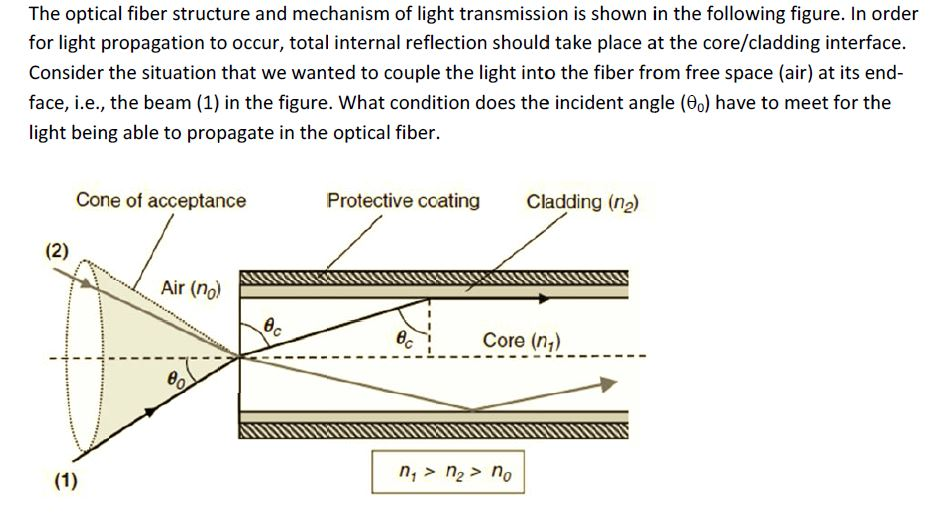The image is a detailed diagram of an optical fiber structure, illustrating the mechanism of light transmission. The diagram includes labeled components such as the core, cladding, protective coating, and the cone of acceptance. The core and cladding are essential parts of the fiber where light propagation occurs through total internal reflection at the core-cladding interface. The figure depicts a cylindrical cone on the left side, indicating the entry point of the light beam into the optical fiber from free space (air). This cone transitions into a rectangular tunnel, representing the fiber. The protective coating and cladding are depicted with black and white striped lines and thin tan lines respectively, while the core is labeled inside the rectangle. The accompanying text at the top of the diagram explains that for light to propagate through the optical fiber, the incident angle must satisfy certain conditions, specifically mentioning the symbols for indices of refraction \(n1 > n2 > n0\). Also visible are related equations crucial for understanding the propagation conditions. The image highlights the importance of the angle of incidence and total internal reflection in the efficient transmission of light through the fiber.